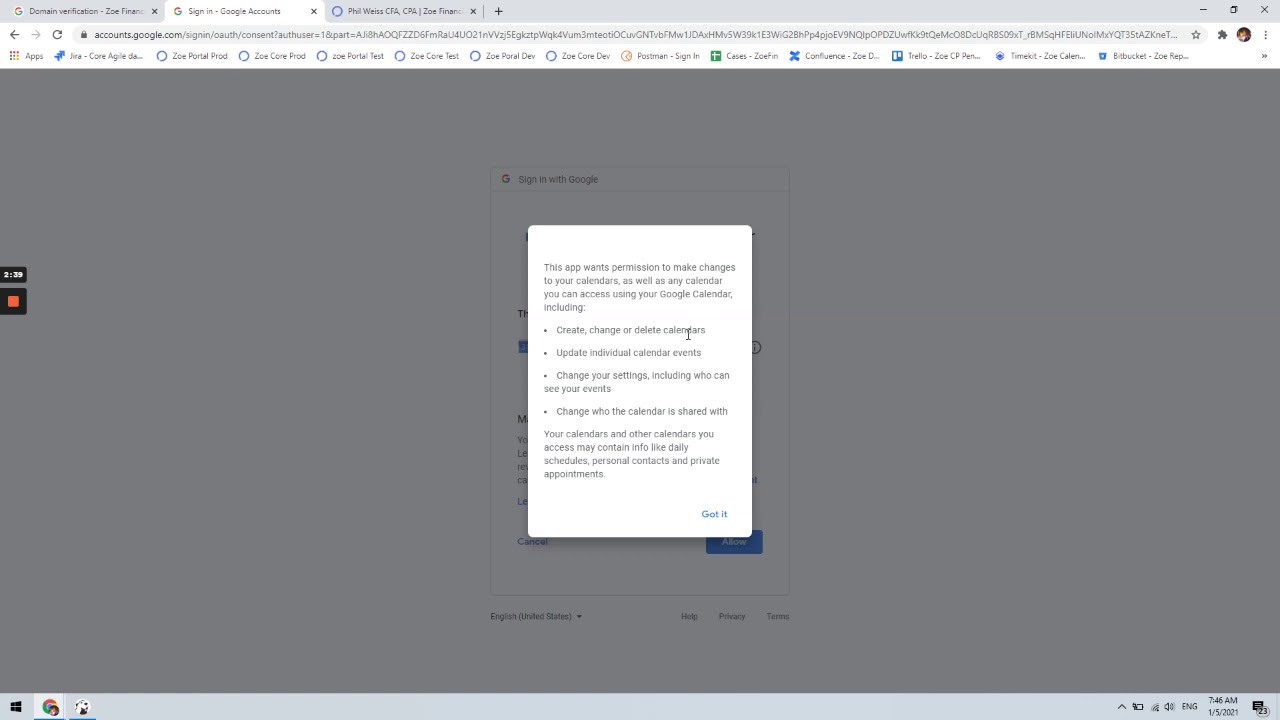The image is a screenshot of a web browser opened to a Google account sign-in page. The main focal point is a smaller, centered white dialog box asking for permissions related to Google Calendar. The dialog box contains text that states, "This app wants permission to make changes to your calendars as well as any calendar you can access using your Google Calendar, including creating, changing, or deleting calendars, updating individual calendar events, changing your settings, including who can see your events, and changing who the calendar is shared with." At the bottom of this dialog box, additional information explains that your calendars and other calendars you access may contain data like daily schedules, personal contacts, and private appointments.

The background behind the dialog box is dim and dark gray, displaying the partially blurred Google login elements. At the top of the browser, three tabs are visible: two are associated with Google, and the third is labeled "Phil Willis CFA," suggesting it may be a financial website.